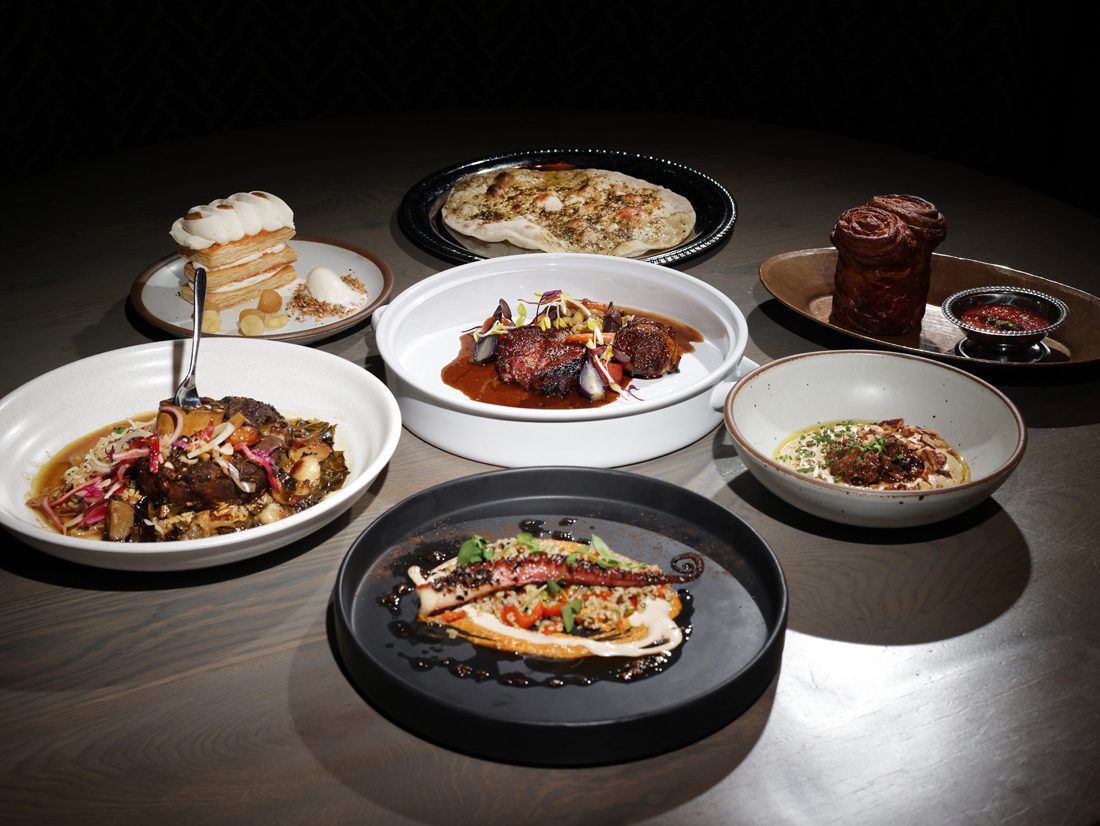The image depicts a dark brown wooden table adorned with seven distinct plates of food, each offering a unique culinary delight. Dominating the forefront is a round, black iron platter featuring a beautifully grilled piece of fish garnished with herbs, complemented by a bed of rice. To its left, a white china plate holds a hearty mixture of noodles and meat, with a spoon ready for serving. Directly behind is a small white dessert plate, showcasing an exquisite white cake with layers of white frosting and a medley of fresh fruits. Centered among the arrangements is a plate of succulent beef medallions, topped with fresh greens. The background features several other intriguing dishes: one plate holds grilled naan bread, while another—a pottery bowl with a brown rim—contains creamy grits adorned with crispy bacon. Finally, an oval brown plate displays two bread rosettes, accompanied by a small round dish of tangy red sauce. Overall, the spread appears varied and rich, perfect for a lavish dining experience or a feature on a culinary website.